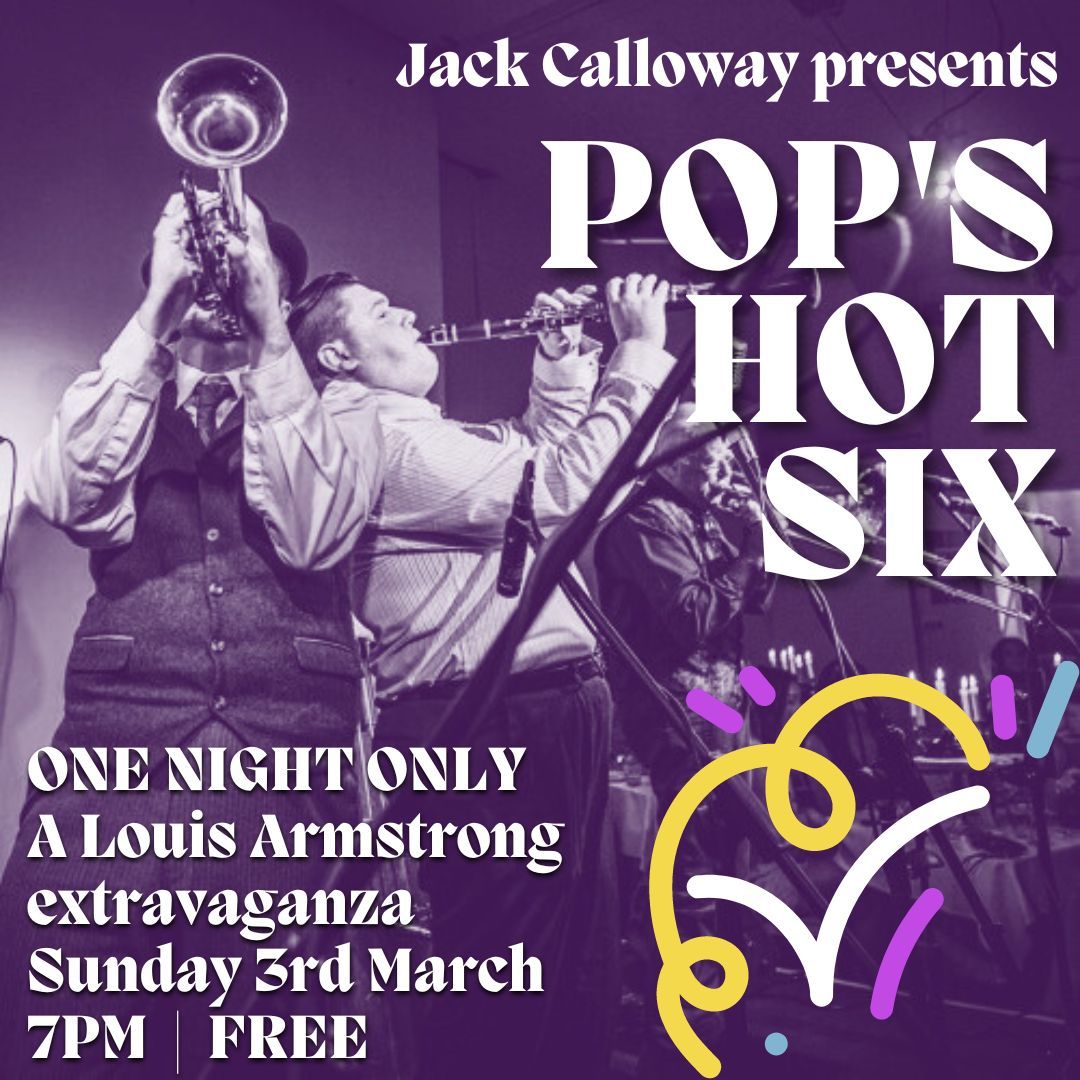The advertisement image showcases a vibrant concert poster for an event titled "Jack Calloway presents Pops Hot 6." The backdrop is a black-and-white photograph with a striking purple tint, featuring three musicians captured on stage. To the left, a man holds a trumpet obscuring his face, while another musician leans back-to-back against him, playing a clarinet. Behind them stands a trombone player, each musician equipped with microphones. The text on the poster highlights the details of the event: "Jack Calloway presents Pops Hot 6" in prominent letters at the top right. Below, in slightly smaller text, it states, "One Night Only – A Louis Armstrong Extravaganza, Sunday, 3rd March, 7pm, Free." Adding a splash of color, the bottom right corner is adorned with decorative squiggles and lines in yellow, white, and purple hues.